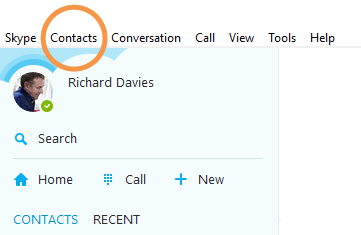The image is a screen capture of a software application, likely Skype, as indicated by the navigation tabs at the top. It is a small, horizontally rectangular image with a white background. Dominating the lower left portion of the frame is a pale blue rectangular section featuring a user profile for Richard Davies. His circular avatar, positioned to the left within this section, depicts a light-skinned man with short dark hair, dressed in a dark shirt or jacket. A small green check mark appears at the lower right of his avatar, signifying his online status.

Below Richard Davies' avatar and name, there are several navigation buttons labeled: search, home, call, new, contacts, and recent. The top navigation bar includes tabs reading Skype, contacts, conversation, call, view, tools, and help, with the 'contacts' tab circled in orange for emphasis. The primary colors in this image consist of white, light blue, sky blue, light green, orange, and black text, creating a clean and user-friendly interface.